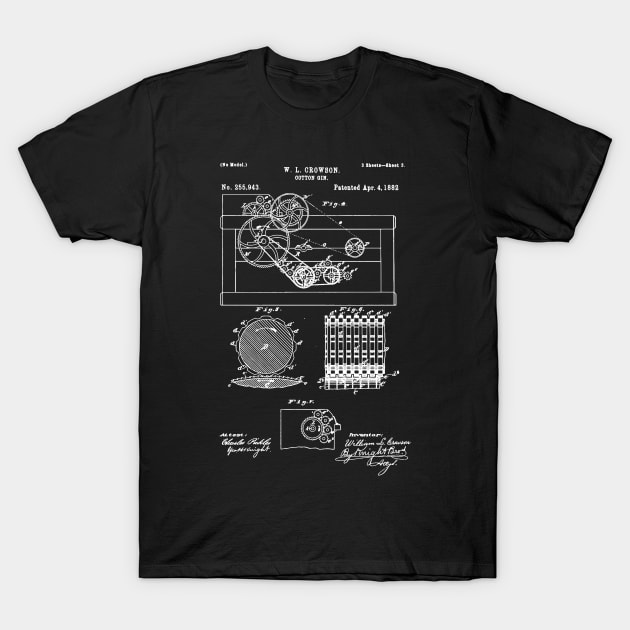This image features a solid black t-shirt with a scoop neck displayed against a white background. The t-shirt is adorned with intricate white graphics and text, primarily displaying industrial blueprints and diagrams related to a mechanism identified as a cotton gin. At the top, the text reads "no model, number 355.943, W. L. Croson, cotton gin," followed by "patent April 4th, 1882." Below this header, an elaborate diagram of the cotton gin is presented, showcasing various interconnected gears and mechanisms. Additional diagrams, including circular and engine-like components, are spread across the shirt. Despite the detailed illustrations, the small white cursive text and some portions of the graphics remain largely illegible. The overall design looks like engineering schematics, offering a vintage, technical aesthetic to the garment.